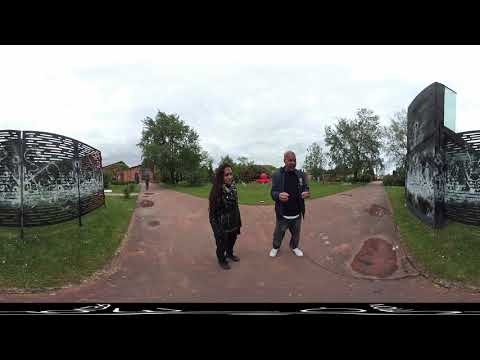This is a slightly distorted panoramic image of two people standing on a brown pathway that splits into two walkways leading off into the horizon. The individuals' proportions appear altered, with short legs and elongated torsos. On the left is a woman with dark skin, long dark hair, and dressed in all dark clothing, including a long-sleeve top. On the right is a man with dark skin, wearing a long-sleeve jacket, dark pants, and white tennis shoes, with a glimpse of a white t-shirt underneath. The man appears to be holding something in his left hand and gesturing with his right hand as he talks. The setting features metal structures on both sides—on the far left, a thin, see-through metal wall in the grass, and on the right, a circular metal structure with black and white patterns. The background includes houses, expansive grassy areas, and trees under a light blue sky.